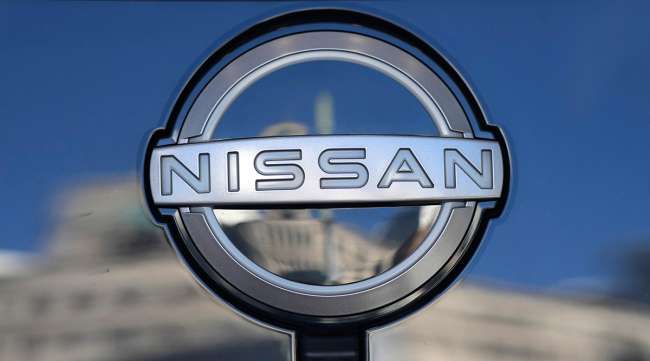This is a detailed close-up photo of a Nissan automobile emblem. The emblem, marked by its signature brand name "NISSAN," is metallic silver, circular in shape, with a broad band running horizontally across its center. The word "NISSAN" is clearly etched in the middle of the band. The background of the image is a bright blue sky, likely midday, with a faint reflection of a government building visible on the highly polished surface of the car, suggesting the emblem may be on a gas cap rather than the hood due to a noticeable space at the bottom for lifting. The emblem itself appears to be reflective, capturing the surrounding environment, adding depth to the overall image.